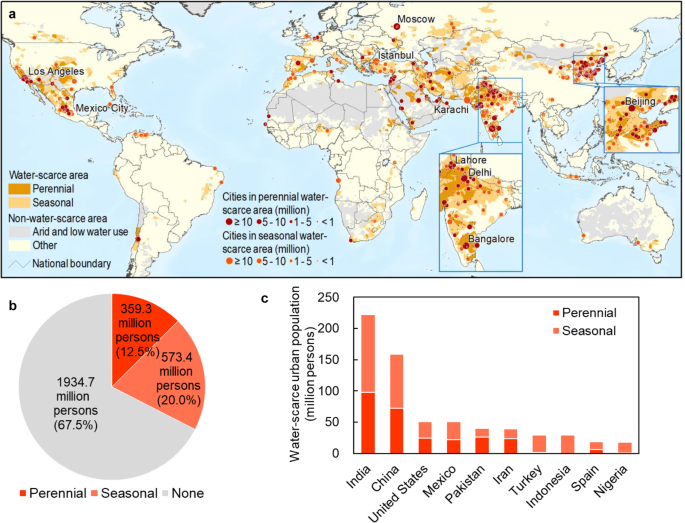This detailed map of the world highlights areas affected by water scarcity, with a focus on India and parts of China. It is color-coded to indicate regions of water scarcity: orange represents perennial water scarcity, while a light orange to dark yellow gradient signifies seasonal water scarcity. Regions that are not affected by water scarcity are shown in white and gray. 

In the bottom left corner, there is a pie chart showing the global population affected by different types of water scarcity: 359.3 million people face perennial water scarcity, 573 million people experience seasonal water scarcity, and 1.9 billion people do not face water scarcity. 

Additionally, a bar graph presents a breakdown of affected populations in eight countries: India, China, the United States, Mexico, Pakistan, Iran, Turkey, Indonesia, Spain, and Nigeria. The map effectively illustrates the severe impact of water scarcity and highlights the regions and populations most affected by this critical issue.